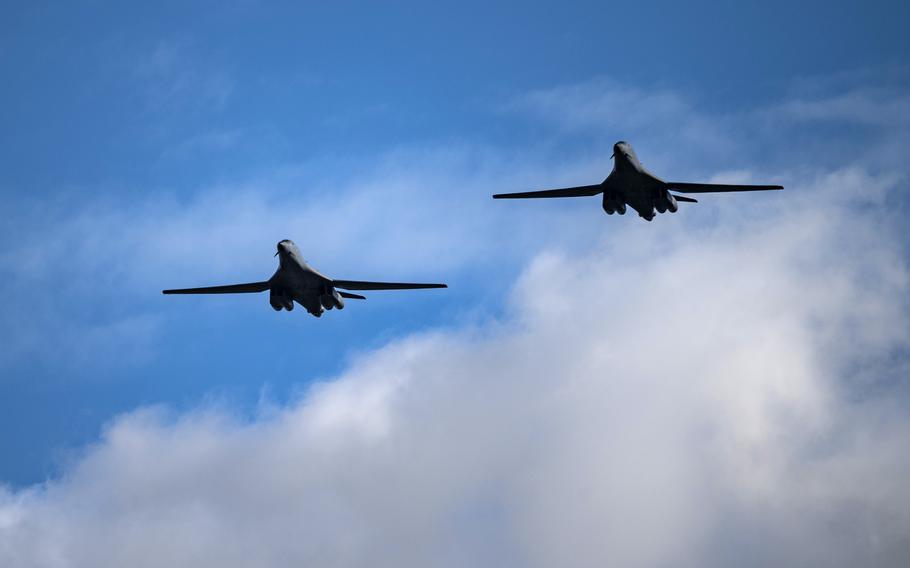In this detailed photo, two gray military jets are captured flying in close formation against a vibrant blue sky. The jets, distinguishable by their long, straight wings and four rear-mounted jet engines, seem identical and are both positioned above a panorama of puffy white and slightly gray clouds. The jet on the right is slightly ahead and higher than the one on the left, and both are largely viewed from below, their undersides cast in shadow due to the sunlight coming from the upper right of the image. The planes exhibit bird-like features, with extended wings and protruding noses, contributing to their sleek, agile appearance. It is daytime, as evidenced by the bright blue backdrop and the sharp clarity with which the jets and clouds are depicted. Despite appearing in flight, the jets maintain a steady and level orientation, almost gliding through the serene, expansive sky.